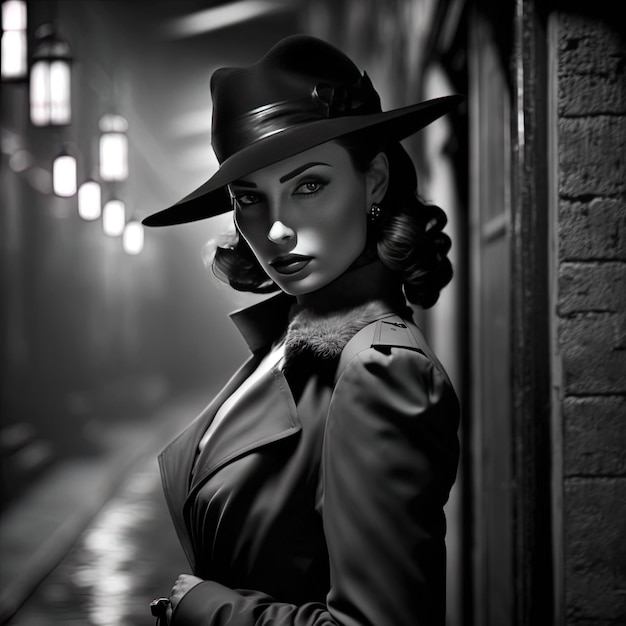A detailed black-and-white photograph, evocative of film noir, capturing a woman in a nighttime alley setting. She stands facing a brick wall with a side view, her left side turned towards the brick backdrop while her face, with its expressive and curved eyebrows, displays a serious expression as she looks directly at the viewer. Her shoulder-length hair cascades in curls, particularly at the ends, framing her composed face accentuated by lipstick. She carries an air of vintage sophistication, wearing a dark wide-brimmed hat and a long coat with a fur collar, which appears as a grayish hue in the monochromatic palette of the picture. The photograph's atmosphere is further enriched by the blurred, shiny surface of the left side of the alleyway, suggesting wetness, likely from rain. Illuminated lanterns affixed to an indistinct building stretch down the alley, adding a subtle, glowing light that punctuates the otherwise moody and grayscale scene, reminiscent of late 1940s or early 1950s cinematography. Despite the computer-generated perfection of her features and attire, which lends an almost surreal quality to the image, her presence is distinctly emotive and engaging amidst the picturesque, rain-kissed urban setting.